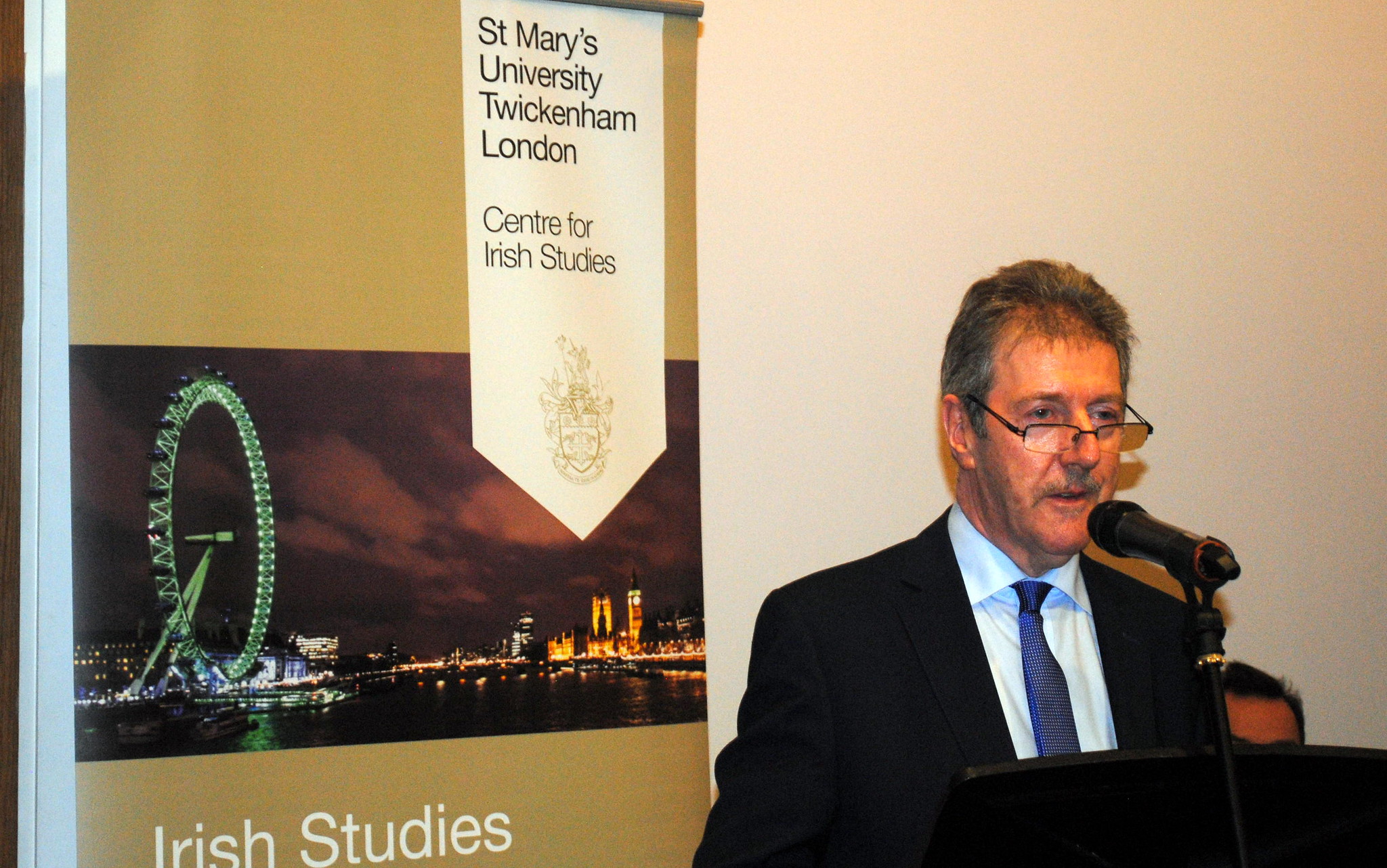In the image, an older man, likely in his 50s or 60s, is speaking into a black microphone at a dark podium. He has short dark and silver hair, glasses perched low on his nose, a mustache, and is dressed in a dark blue suit jacket, white shirt, and a blue tie. Behind him is a large, illuminated banner that reads "St. Mary's University, Twickenham, London Center for Irish Studies," featuring a detailed image of London’s skyline, including the iconic Big Ben and the London Eye Ferris wheel, both lit up against the evening sky. The banner also has a coat of arms and the words "Irish Studies" prominently at the bottom. To the lower right, just behind the speaking man, there is another seated man, whose presence is only indicated by the visible top of his glasses, forehead, and hair.